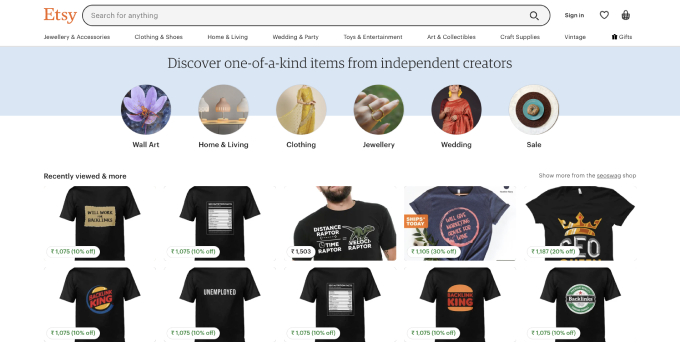The image displays the Etsy homepage, featuring the iconic orange "Etsy" logo prominently at the top. Below it, a search bar is centered, flanked by options to sign in, a heart symbol representing favorites, and a lock symbol for secure transactions. The site's main navigation menu is visible, listing categories such as Jewelry & Accessories, Clothing & Shoes, Home & Living, Weddings, Parties, Toys & Entertainment, Art & Collectibles, Craft Supplies, Vintage items, and Gifts.

Beneath the navigation menu is a light blue rectangular box overlaid with the text: "Discover one-of-a-kind items from independent creators." This section is accompanied by six circular icons each representing a different category: Wall Art, Home & Living, Clothing, Jewelry, Weddings, and Sale, each illustrated with a relevant profile picture.

Further down, the page highlights a "Recently Viewed & More" section. This section is organized into two rows, each displaying five different t-shirts with their corresponding prices clearly marked beneath each item.